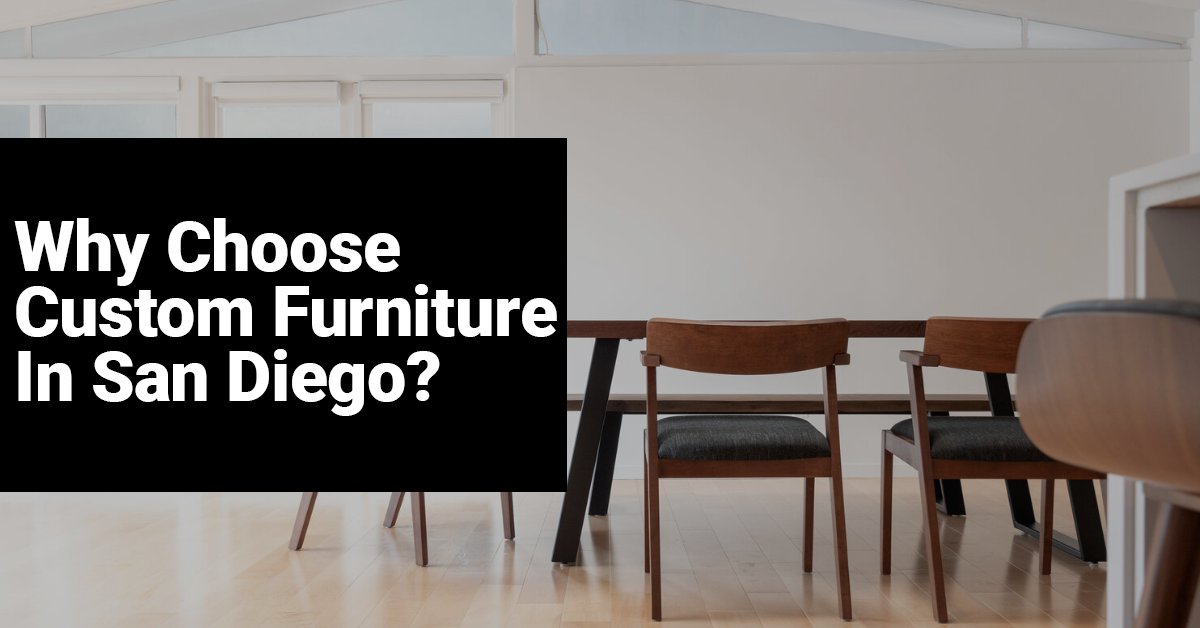The image features a modern dining room setting with a wooden-topped table that has sleek black legs. Surrounding the table are four chairs characterized by their wooden backrests, thin wooden legs, and black cushioned seats. The chairs, which do not have armrests, feature a distinctive design with thin, curved, rectangular back pieces. The room has a clean and minimalist aesthetic, highlighted by beige walls and a wooden floor, adding a warm and inviting feel to the space. On the left side of the image, a prominent black rectangular sign displays white text reading, "Why Choose Custom Furniture in San Diego?" There are no additional decorations on the walls or table, further emphasizing the furniture as the focal point of the image. The photograph captures a horizontal, rectangular layout, and a simple doorway is visible to the right.